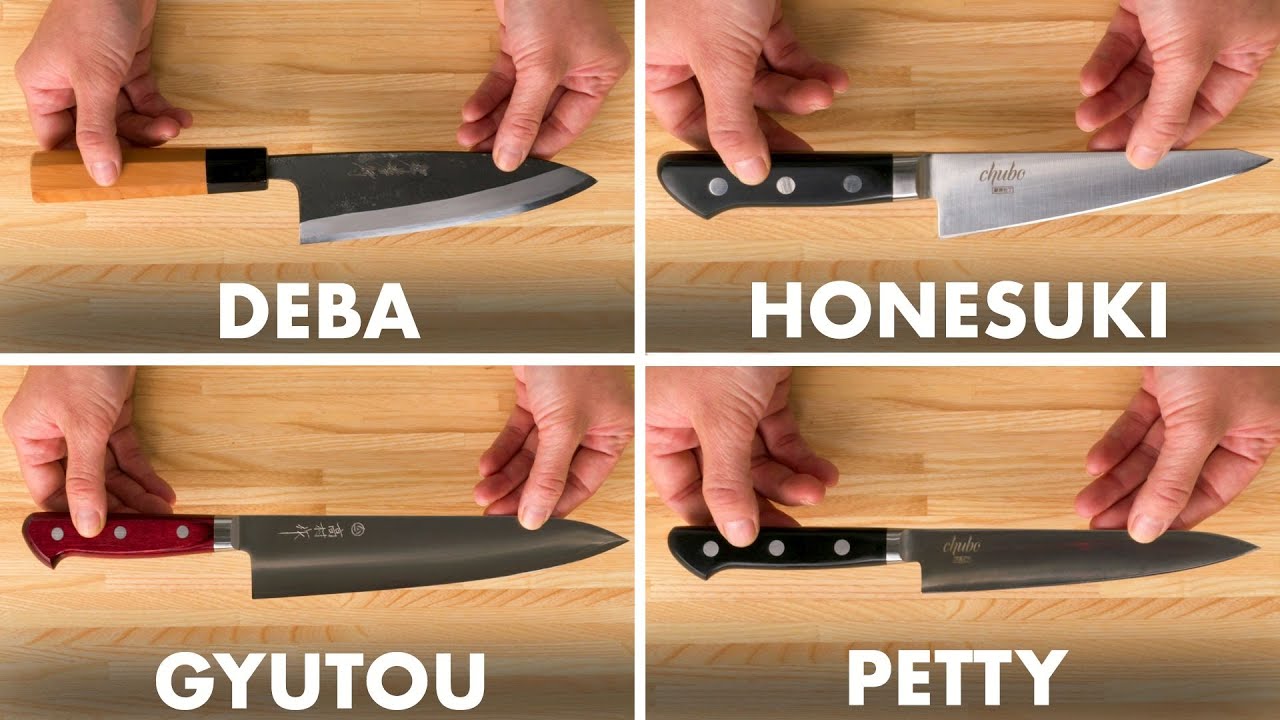The image is divided into four connected rectangular panels, each displaying a different type of knife positioned on a wooden surface. The knives are held by a pair of white-skinned hands, with both thumbs visible on top of the knives in each panel. The knives are oriented with their blades pointing to the right.

**Top Left Panel (Deba):** The knife, labeled "DEBA" in thick white capital letters, features a brown, octagonal handle. It has a distinct black section at the top where the blade inserts. The blade is wide and thick, with some engraved text. 

**Top Right Panel (Honesuki):** This knife is labeled "HONESUKI" in white capital letters. It has a black handle adorned with three silver circles and a blade with a triangular shape that includes engraved text. There's also an inscription possibly starting with "CHUBE."

**Bottom Left Panel (Gyutou):** Labeled "GYUTOU" in white capital letters, this knife has an amber-red handle with three silver circles. The long blade is suited for vegetable cutting and features multiple symbols, potentially in a foreign language.

**Bottom Right Panel (Petty):** The knife is labeled "PETTY" in white capital letters. It sports a black handle, also featuring three silver circles, and has a smaller blade akin to a paring knife. Similar to the Honesuki, the blade may have an inscription starting with "CHUBE."

The shared colors across the image include flesh tone white, brown, black, silver, red, and white letters. Each knife shows slight variations in handle color and blade shape but maintains a consistent presentation style.